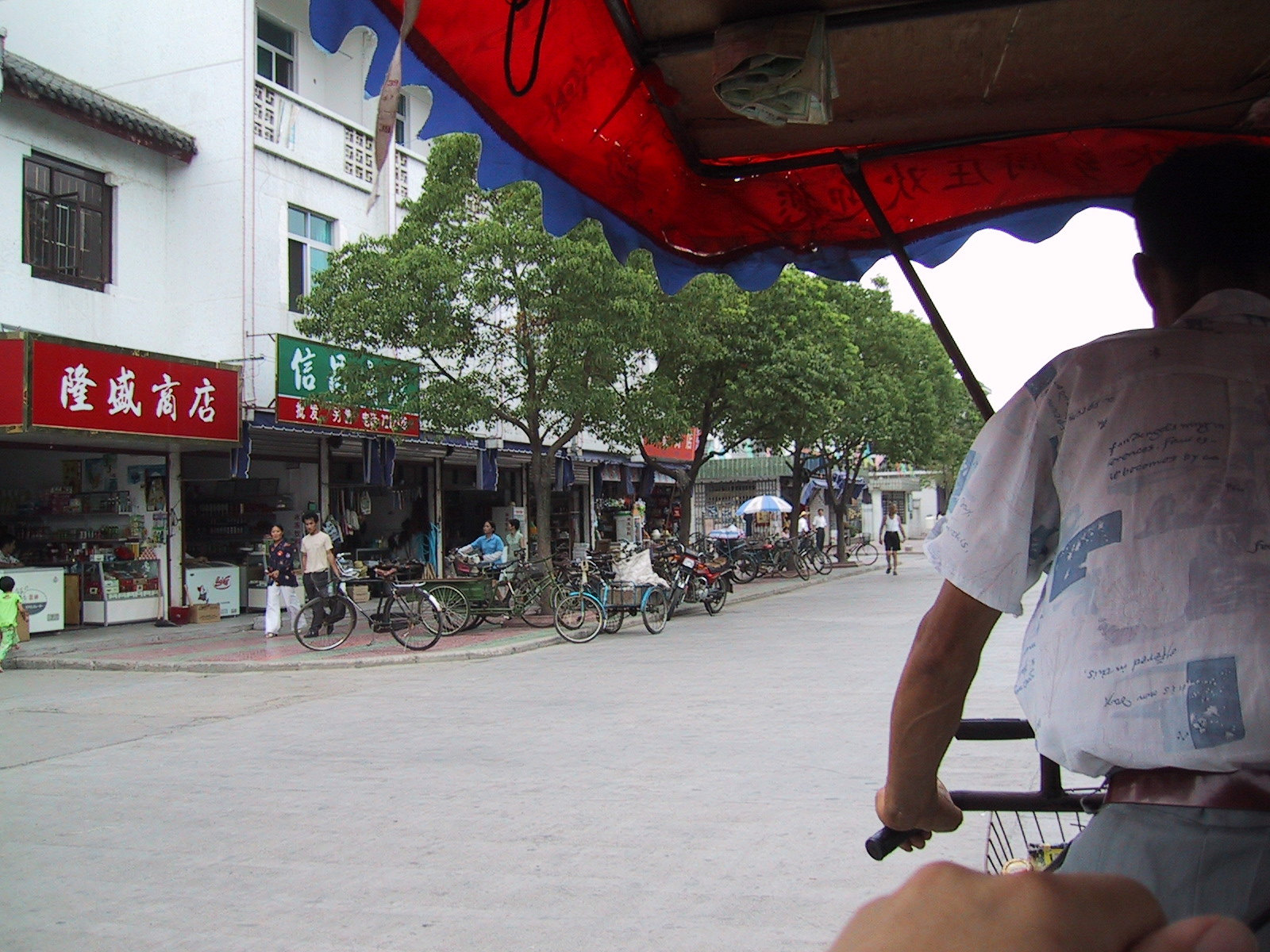A photograph captures a bustling, broad commercial street, likely situated in Asia due to the visible Mandarin characters on the storefronts. The scene is set outdoors on a gray cobblestone street under an overcast sky, adding a muted tone to the vibrant neighborhood. Tall, multi-story white buildings frame the scene, their open, small business-oriented shops lining the sidewalks without doors or windows, creating a sense of accessibility and openness.

In front of these shops, a varied collection of parked bicycles and mopeds hints at the preferred mode of transportation. Mingling pedestrians stroll along the sidewalks, creating a sense of community even though the street itself is devoid of cars. Sparse trees with green leaves punctuate the sidewalk, providing a touch of nature amid the urban setting.

The photograph is taken from the perspective of a passenger in a group bike taxi service, identified by the visible right hand of the driver in a short-sleeved shirt, brown belt, and shorts. The photographer's own hands appear in the lower right corner of the image, further adding to the immersive, candid feel. This commercial district, teeming with subtle life, offers a glimpse into the daily rhythm of the area, whether it is a neighborhood in the Far East or a vibrant Chinatown located elsewhere in the world.